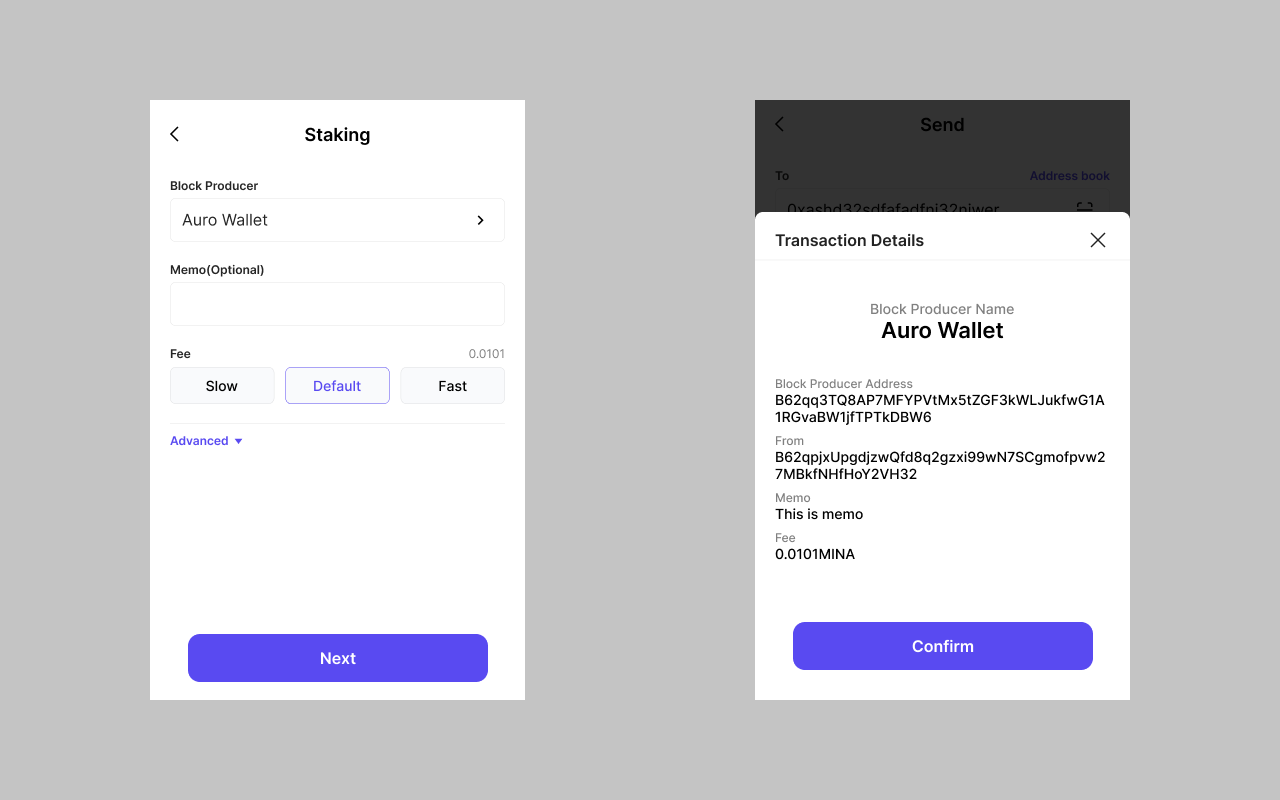The image features a light gray background with two vertically oriented rectangular boxes side by side.

The left box, set against a white background, displays a '<' symbol in the top left corner. To its right, the word "Staking" is prominently written, with "Block Producer" located beneath it. Below this, there is an interactive dropdown box labeled "Euro Wallet," allowing users to switch between options. Further down, the phrase "Memo (Optional)" is present, accompanied by a text field for user input. A section labeled "Fee" follows, featuring three selectable options: "Slow," "Default," and "Fast." Below these settings, a blue hyperlink labeled "Advanced" is available for more detailed configurations. At the bottom, a blue button marked "Next" prompts users to proceed with the process.

The right box, distinguished by a black border at the top, also has a white background. It is titled "Transaction Details" and contains several fields: "Block Producer Name," "Euro Wallet," and "Block Producer Address," with the latter accompanied by the specific address "B62QQ3TQ8A."

Overall, the image comprehensively details the user interface for managing staking and transaction configurations within a cryptocurrency application.